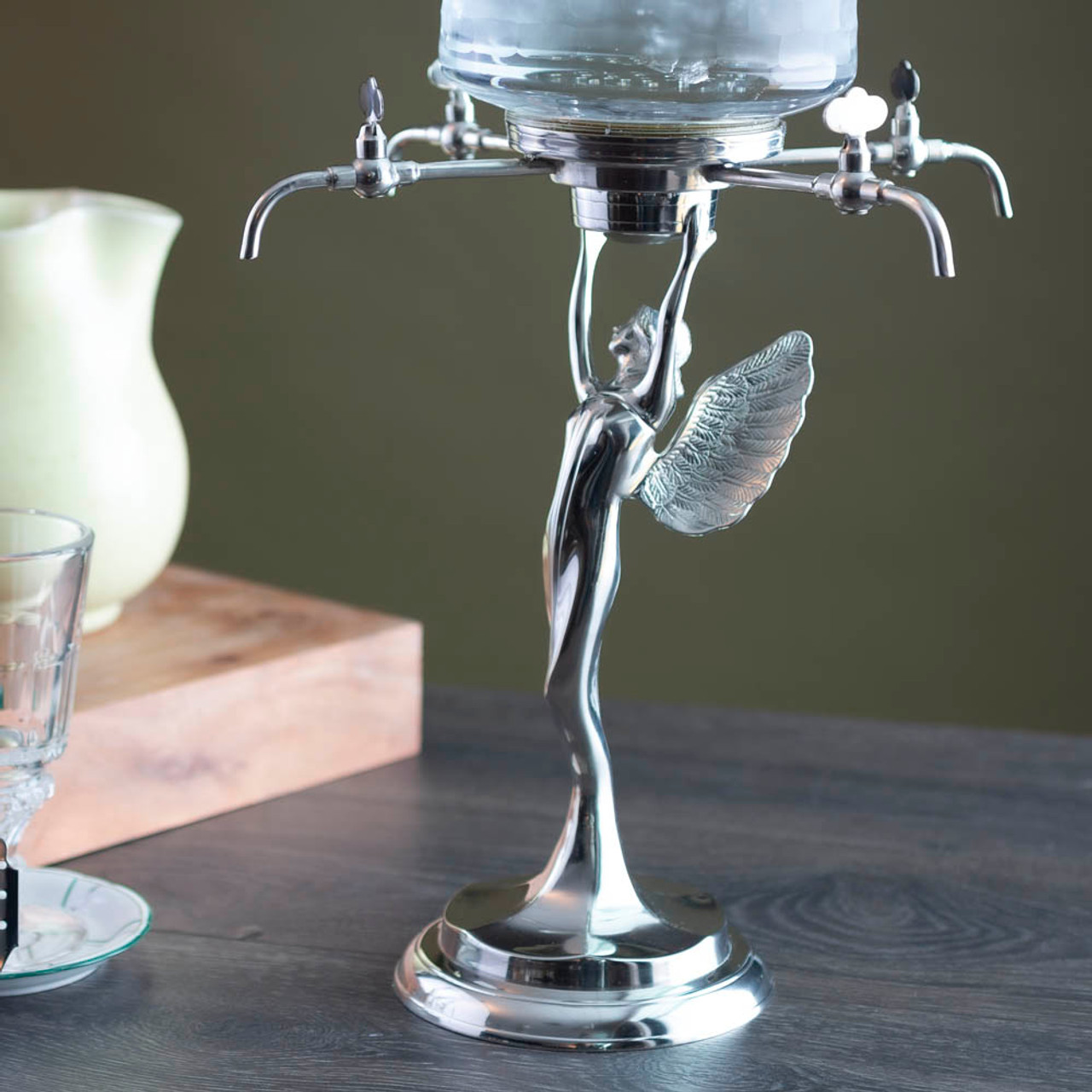This photograph showcases a unique liquid dispenser standing on a dark gray wooden table. The central feature is a silver statue of a tall, skinny angel with one visible wing and outstretched arms, holding up a glass container filled with clear liquid. The container rests on a silver base resembling a trophy and has four silver spouts protruding from the bottom. Surrounding the dispenser, on the table, there's a glass jar positioned to the left, and nearby, a small clear glass and a dish. In the background, a copper platform holds a white vase, and there appears to be a wooden cutting board. The intricate design and the meticulous details of the statue and the dispenser make it a captivating centerpiece.